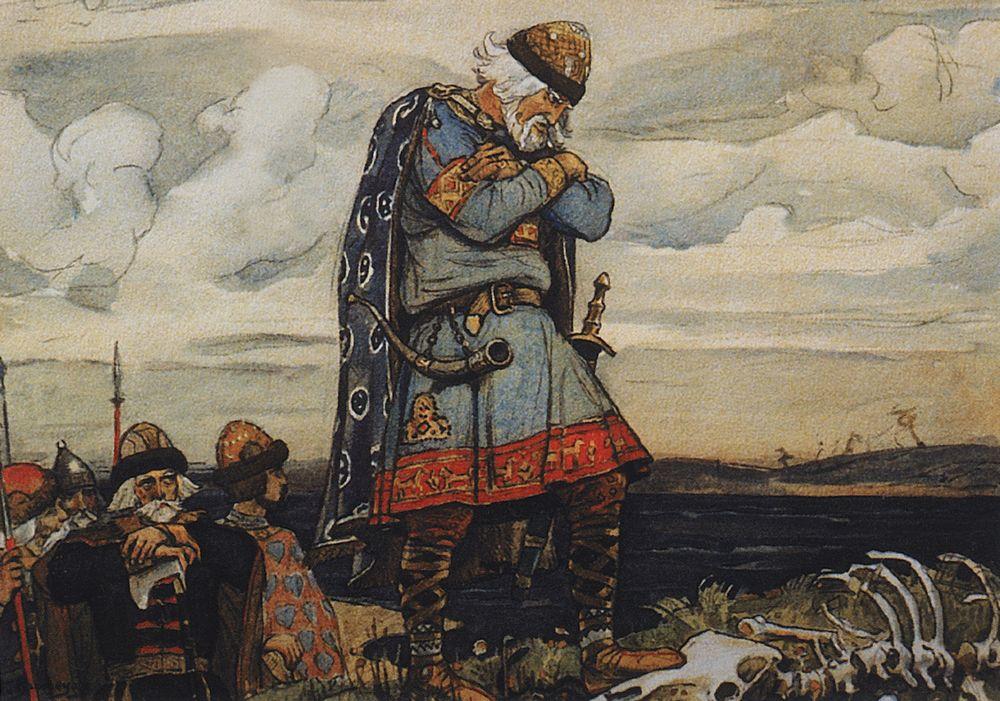The painting depicts a somber Viking in a dynamic, medieval scene. The central figure, an older man with coffee-brown skin, has white hair that falls past his ears and a white beard and mustache. His facial expression is serious, possibly upset, and he is looking down at the ground. He wears a distinctive cap with a goldish-brown rim and a lighter brown top. He's dressed in a blue robe featuring intricate red trim and a blue and white cape. Around his waist, he's fastened a belt that holds a Viking horn on a chain and the scabbard of a sword. His legs are wrapped in leather, and he's wearing lace-up boots that rise to his knees. The man appears to be standing on a field scattered with animal bones, with one foot atop part of a skeleton.

Behind him, a gathering of soldiers similarly clad in different colored robes and identical hats can be seen. One soldier stands with his hands folded across his chest, while others hold spears. The landscape is bleak and gloomy, featuring a dark, possibly battle-scarred ground, transitioning from black soil to a tan terrain. The background reveals rolling hills, a body of water, and a cloudy sky, adding to the melancholic atmosphere of the scene.